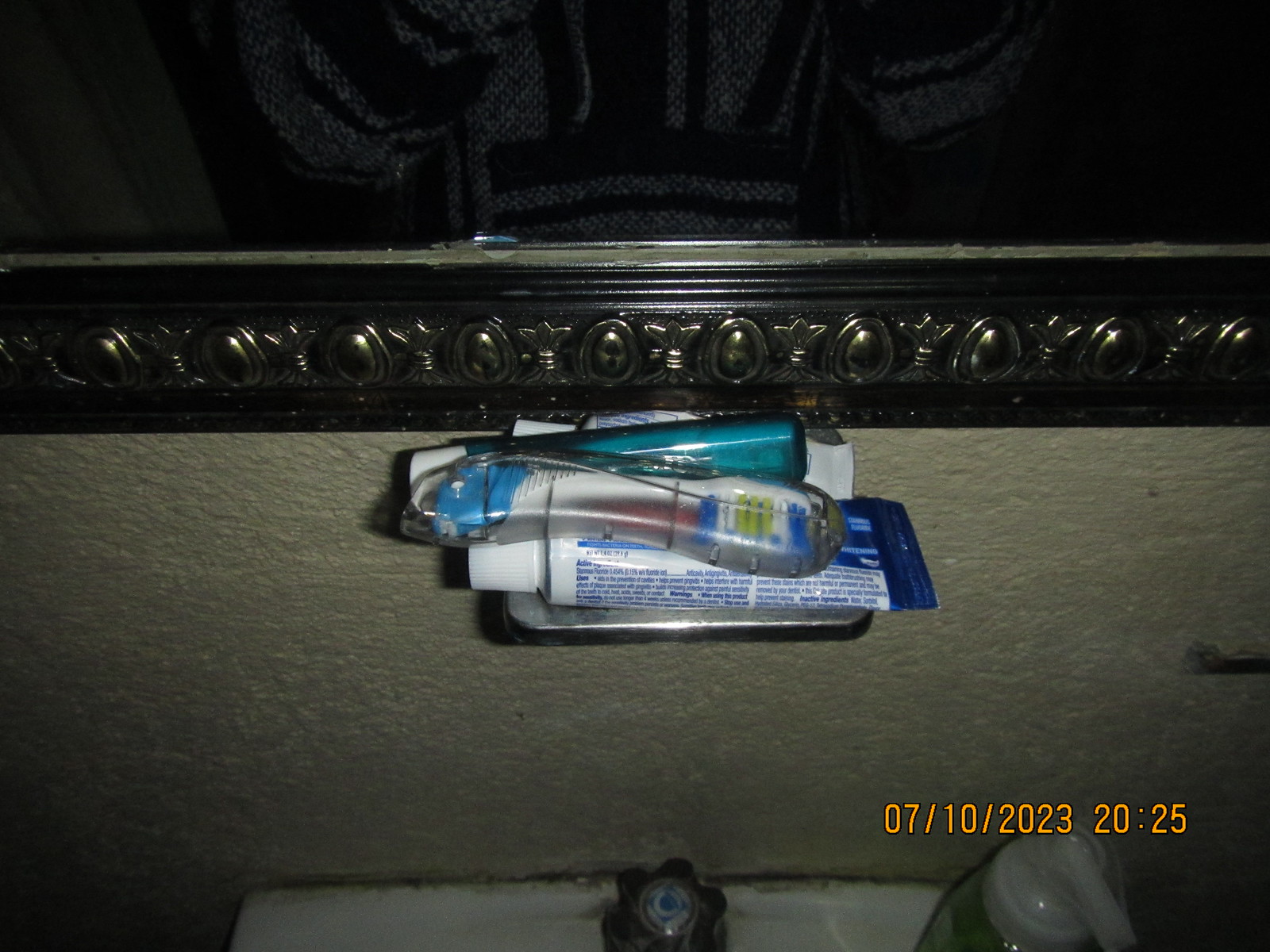This image, set in a bathroom, captures a scene with various elements detailed in a clear snapshot. At the bottom, there's a slightly grimy, white sink featuring a silver handle in the center and a soap dispenser to the right. Above the sink, a small metallic shelf juts out from a grayish wall, holding an assortment of hygiene items: notably, two travel-size toothbrushes—one of which is folded into a clear case—as well as a small tube of toothpaste. 

The upper part of the image showcases a mirror with a decorative metal frame, exhibiting a mix of floral and egg-like patterns. The reflection in the mirror reveals the mid-torso of the photographer, who is wearing a dark, long-sleeved sweater. In bold orange, the digital timestamp "07-10-2023 20:25" is visible in the bottom right corner, indicating the date and time the photograph was taken. The overall ambiance of the image is somewhat dark, contributing to the discernible but shadowed details throughout the scene.